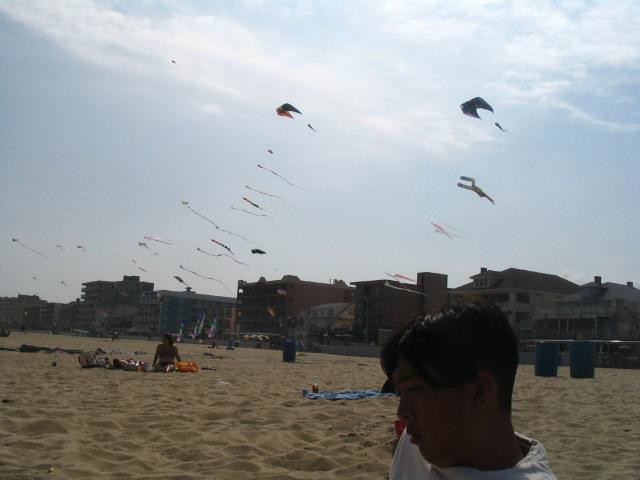The photograph captures a bustling beach scene filled with detailed elements. The sandy beach is dotted with various colored towels, including a prominent blue one close to a man with short black hair and a white collar, standing near the foreground in shadow. This man has dark skin and is looking downward. Just beyond him, another blue towel is visible. To the left and further down the beach, a person sits next to an orange-red towel with their belongings piled beside them. In the sky above, roughly 25 kites or flags of varying sizes are flying, suggesting a kite-flying contest or event. The kites appear like vibrant strings in the air against a backdrop of a blue sky mixed with wispy and white clouds and some grayish-blue hues indicating a slightly overcast day. The background features a line of houses or hotels, adding to the beach’s lively atmosphere. Scattered across the beach are a few cylindrical trash cans, and the scene is bathed in sunlight despite the cloud cover.